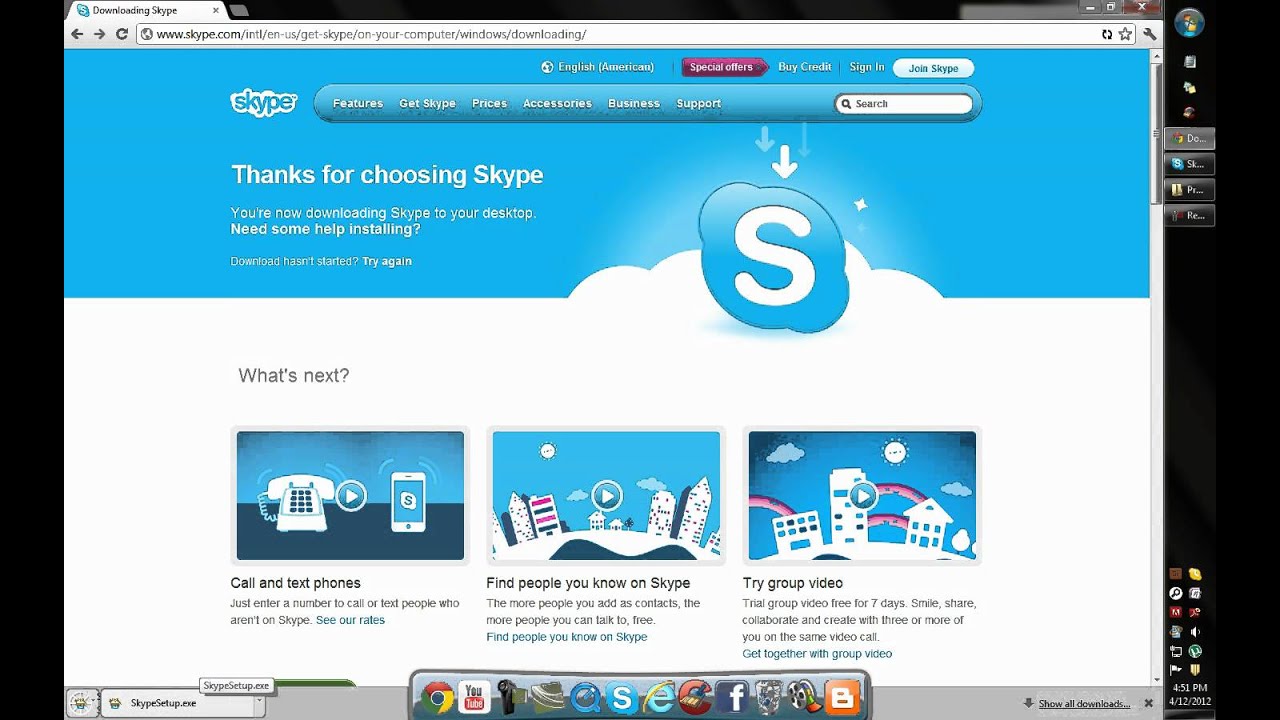A detailed screenshot of a Skype webpage is prominently displayed, capturing the moment when a user is downloading the Skype application to their desktop. The screen features a "Thank you for choosing Skype" message, acknowledging the user's decision to use the service. A progress bar indicates the ongoing download of the Skype Setup.exe file, which is specifically tailored for an English language installation. 

In addition to the download progress, the page offers a range of information and options for the user. It details available special offers from Skype and provides guidance on how to join the platform. Users are prompted to select their intended use of Skype, with options for personal or business purposes. The interface also includes choices regarding payment options and device usage, whether from a phone or computer. 

The page further assists users in connecting with others by explaining how to find people they may know on Skype, initiate a group video call, and other essential features to enhance their communication experience on the platform.